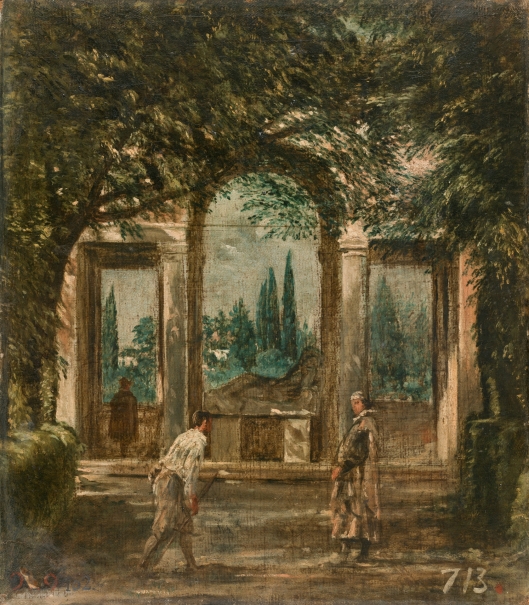The image is a detailed painting that appears to be set outdoors during the daytime, featuring an expansive courtyard or meadow that exudes an antiquated, mural-like quality. In the scene, three men are present within a lush, verdant environment filled with ample trees and bushes both near and in the distant background. The sky, though bright, is not vividly blue or sunny, adding to the aged ambiance of the piece.

On the left, a man equipped with a golf club, donned in a white long-sleeved shirt and light trousers, looks like he has just swung the club. To his right, an older man with white hair is attired in a tan robe. Further back, a third man stands under an open stone or concrete structure with arches and eight white columns supporting a domed top. This man observes the two figures from his vantage point under the arches. The painting's bottom right corner features the white text "713," which might be indicative of some form of signature or annotation. The background reveals more trees and potentially some buildings or homes, enriching the setting with elements of a large manor or estate.